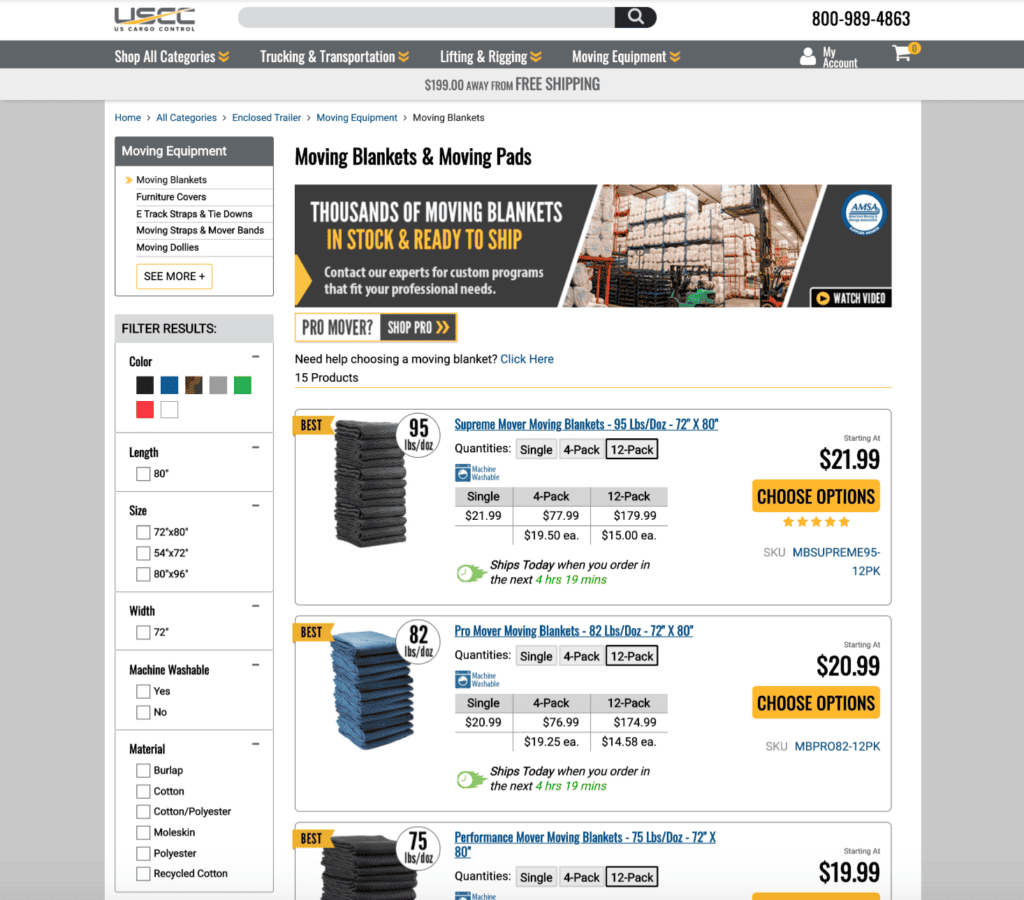The image depicts the U.S. Cargo Control (U.S.C.C.) website with several key sections and elements. 

In the top left corner, a white banner prominently displays the U.S.C.C. initials, likely standing for "U.S. Cargo Control." Adjacent to the right is a gray oval containing a magnifying glass icon, indicative of a search function. Further right, the contact details include a 1-800 number.

Below this section, a horizontal gray banner features several drop-down options labeled "Shop All Categories," "Trucking and Transportation," "Lifting and Rigging," and "Moving Equipment." To the far right of these options, there's a profile icon labeled "My Account," accompanied by a shopping cart icon displaying a notification circle.

Beneath this navigation bar, a secondary gray banner informs users they are "$199 Away From Free Shipping." Directly below, the focus shifts to a section on Moving Blankets and Moving Pads, featuring a highlighted message "Thousands of Moving Blankets in Stock and Ready to Ship," with "in stock and ready to ship" emphasized in yellow.

To the right, a media image shows forklifts operating within a warehouse, highlighting the effectiveness of the moving aids. Further down, on the left sidebar, filtering options for results include categories such as colors, length, size, width, machine washable material, and more, allowing for detailed product searches.

On the right section are three product selections: Supreme Mover Moving Blankets, Pro Mover Moving Blankets, and Performance Mover Moving Blankets, each accompanied by their respective prices. The first product stands out with an apparent customer rating system.

This detailed layout ensures easy navigation and product discovery for users seeking moving and cargo control solutions.